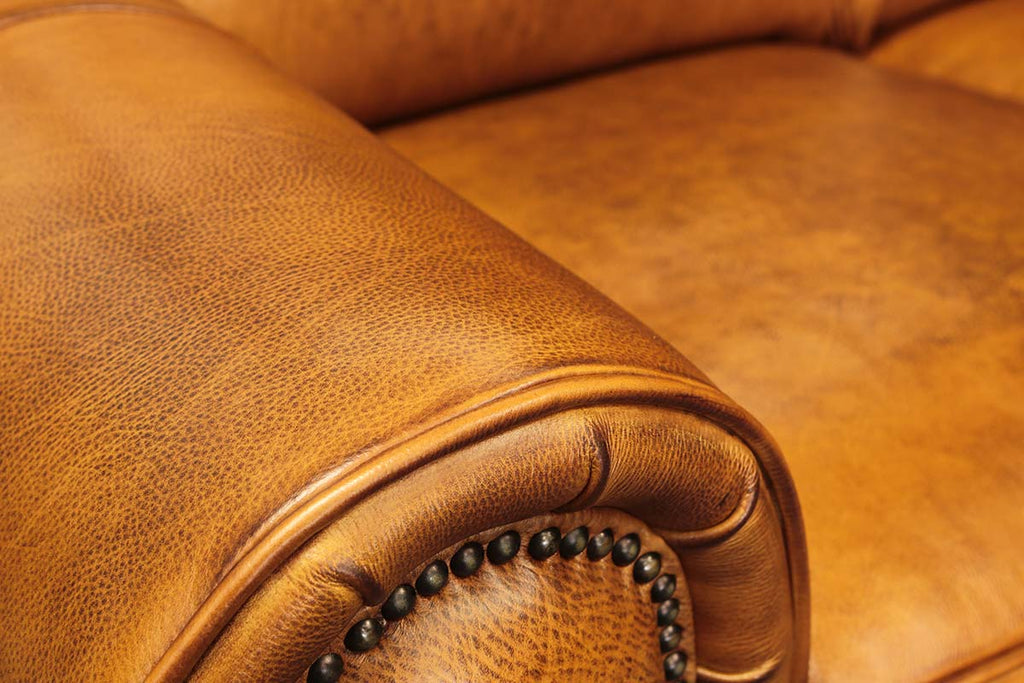The photograph features a detailed close-up of the left-hand side arm of a luxurious leather lounge chair. The chair's rich, smoky brown leather evokes the color of a well-worn baseball glove, suggesting a sense of comfort and timeless use. Adorning the front of the armrest are metal grommets that not only serve a decorative purpose but also add a touch of character and craftsmanship. The image focuses sharply on the arm of the chair, revealing its well-cushioned and inviting texture, while the background blurs slightly to hint at the seat and backrest without drawing attention away from the intricately detailed arm. This worn yet cozy piece, which would be perfectly suited for an old office or library, invites thoughts of relaxation and leisurely reading.